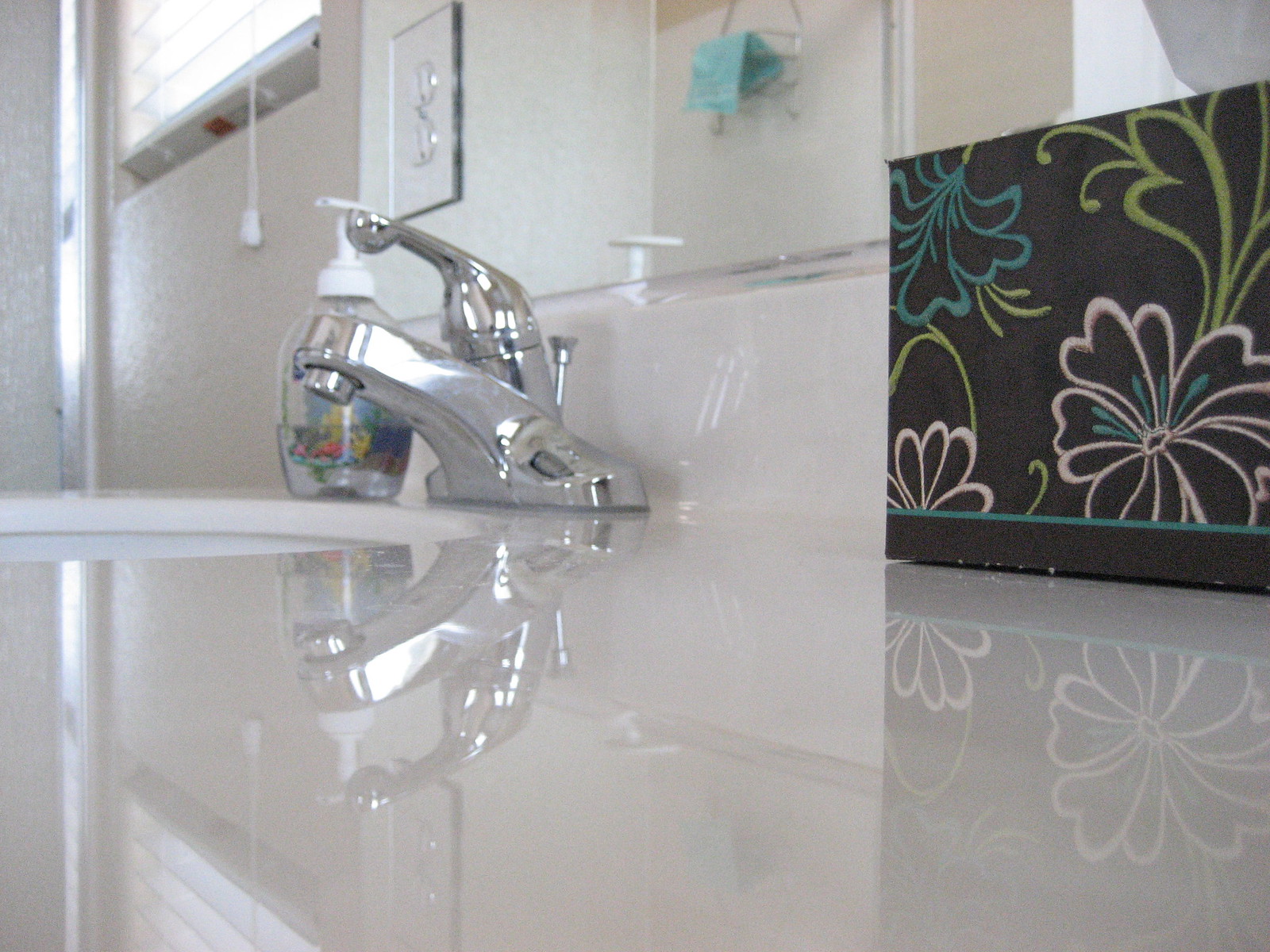A pristine bathroom countertop gleams under the natural light streaming through partially opened blinds. The counter, immaculately clean and highly reflective, showcases meticulous attention to detail. At the center stands a chrome faucet, its sleek design accentuated by the clear reflections on the shiny surface. Nearby electrical outlets, framed by glass, add a modern touch to the scene. To the right sits a black tissue box adorned with floral patterns, its top tissue expertly ready for use. On the left, a hand soap dispenser stands neatly in place. 

Behind the faucet, a large mirror captures and reflects the intricate details of the room: the neat countertop, the tissue box, and even the light filtering through the window. Further in the reflection, an aqua-colored towel hangs tidily on a towel rack, adding a touch of color to the sophisticated setting. The overall ambiance is one of cleanliness and modern elegance, highlighted by the interplay of light and reflections throughout the space.